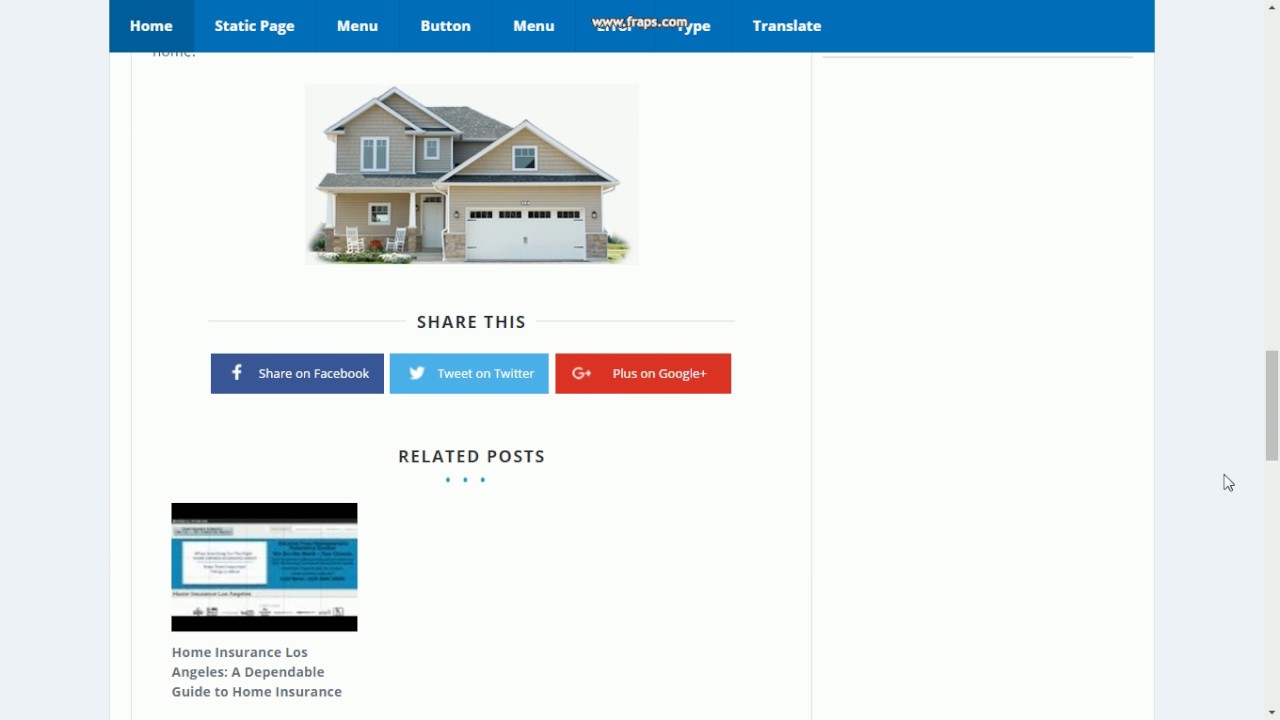Screenshot from www.fraps.com featuring a blue header with menu buttons for 'Home', 'Static Page', and 'Translate'. In the center of the page is an image of a two-story house. Below the image, there are social sharing buttons: 'Share this on Facebook' in a blue rectangle, 'Share on Twitter' in a light blue rectangle, and a 'Google+' button in an orange rectangle. Nearby, a related post is visible titled "Home Insurance Los Angeles: A Dependable Guide to Home Insurance". The website has a white background, and the computer screen's background is light blue. On the right side of the screen, a gray scroll bar is positioned just over halfway down the page.